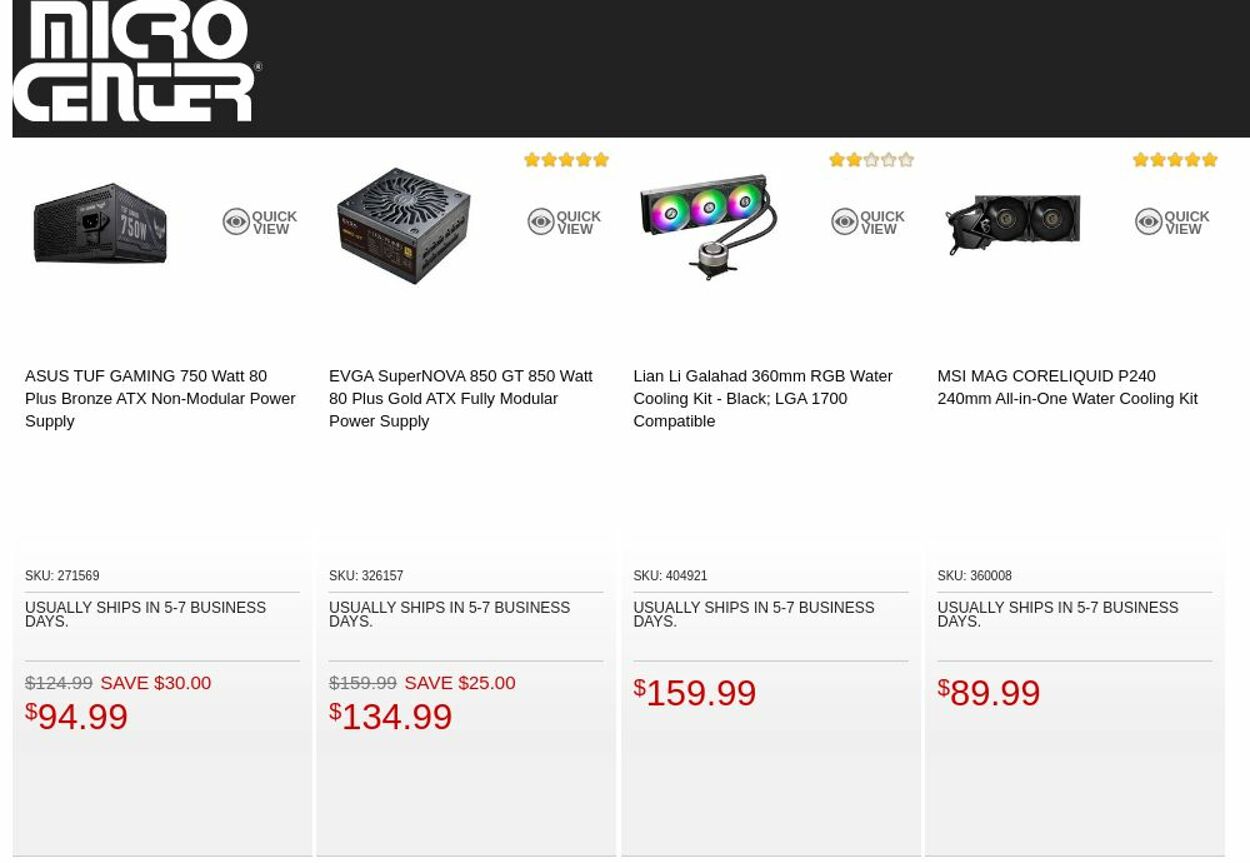The image captures a section of a Micro Center store, identifiable by the store's logo in the upper left-hand corner. The logo features "Micro Center" in a white font, with "Micro" positioned above "Center," all set against a black horizontal bar that spans the width of the image. Displayed prominently are four computer hardware items.

1. On the far left, an **Asus TUF Gaming 750 Watt 80 Plus Bronze ATX Non-Modular Power Supply** is showcased with a price tag of **$94.99**.
2. Next to it is the **EVGA Supernova 850 GT 850 Watt 80 Plus Gold ATX Fully Modular Power Supply**, priced at **$134.99**.
3. The third item, a sleek black cooling kit, is labeled with a price of **$159.99**.
4. The last item is depicted as a core liquid kit, retailing for **$89.99**.

Each item is neatly arranged, making it easy for customers to view the products and their respective prices.